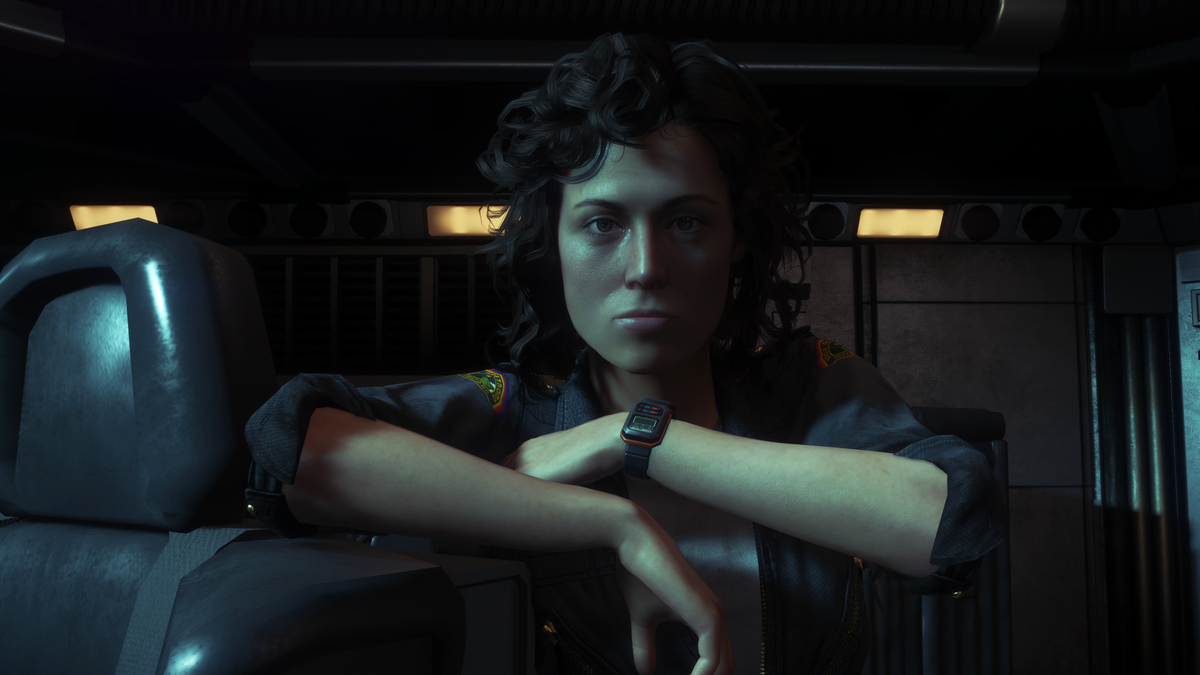The image depicts a highly realistic, computer-generated 3D graphic of a young Caucasian woman with shoulder-length black curly hair. She is dressed in a dark gray to black uniform with sleeves rolled up to her elbows. The uniform features patches on both shoulders and is slightly open at the collar, revealing a gray-white shirt underneath. A black digital wristwatch adorns her left wrist. The woman has a serious expression, with dark eyes and a neutral, straight face. She is leaning forward, elbows crossed, resting her left hand on her right wrist, on a highly padded black leather chair equipped with a black seatbelt strap. The setting appears to be the interior of a large vehicle—possibly a utility armored vehicle or a spaceship—evidenced by the visible black seat, three lights, dark ceiling, gray metallic panels, and steel conduit pipes. The backdrop includes low lights and metallic elements, adding to the industrial or high-tech atmosphere.